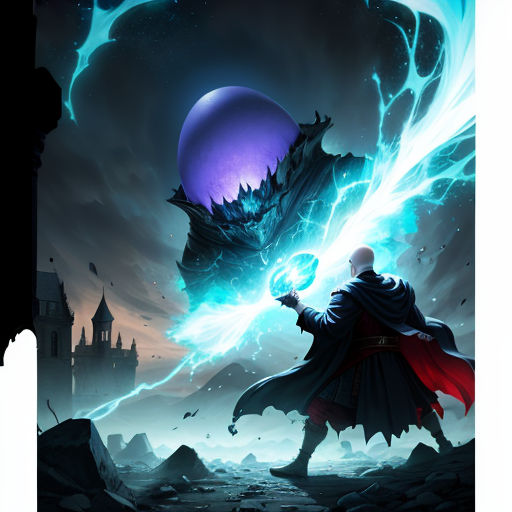This highly detailed, computer-generated vertical rectangular image, reminiscent of a video game cover, depicts a bald man seen from behind, dressed in a long, black trench coat with red lining and black boots. He stands in the lower right corner, his left hand holding a swirling ball of blue and white energy that spills and arcs upwards like water or light. His back faces us, and his gaze is directed towards a large, ominous figure with a round, purple egg-shaped head wrapped in a tattered black mask. The giant figure, suspended in a black and gray overcast sky, looms menacingly above. To the left, the background reveals a desolate, rubble-strewn landscape with a castle tower featuring a triangular roof and other English-style houses. The left side of the image extends outward with a wider black border that has a dripping effect halfway down, adding to the dark and foreboding atmosphere.